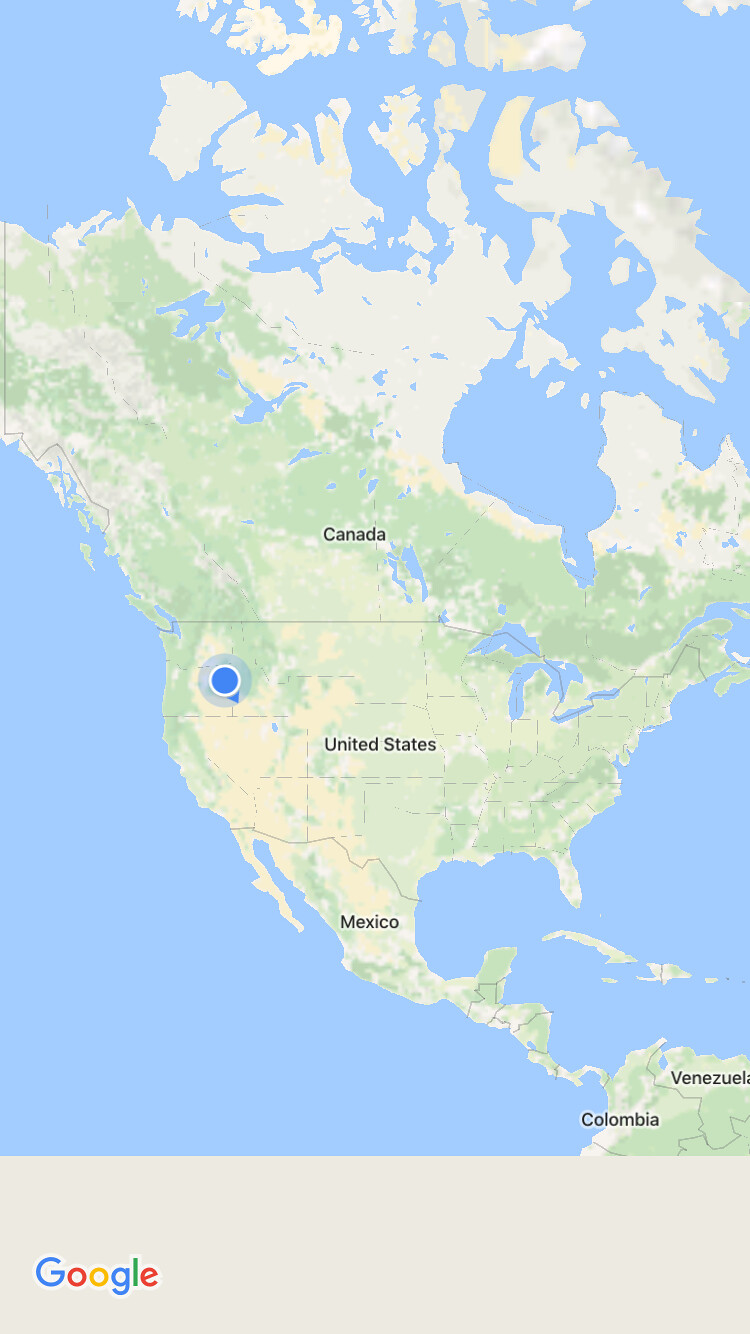The image is a screenshot from a cell phone displaying a Google Maps view primarily focused on North America. The map highlights the United States, Canada, and Mexico in various shades of green, with the waters in blue and northern territories in white. Additionally, the map includes partial views of Venezuela and Colombia at the bottom. A blue dot is located near the Oregon-Washington state border, indicating a specific location in the Pacific Northwest. At the bottom of the image, a beige-colored horizontal bar with the word "Google" in its iconic blue, red, yellow, and green colors, appears on a gray background. The map includes minimal text, showing country names like Canada, United States, Mexico, Colombia, and Venezuela in black.